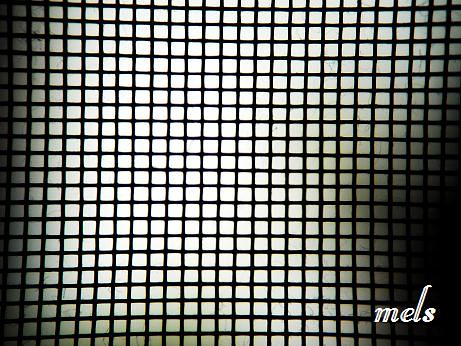The image depicts a minimalist, optical illusion pattern consisting of white and black tiles forming a grid. The white tiles are intersected by black lines, creating an effect where small white circles seem to appear at the intersections of the lines the longer you stare at it. This illusion may be intentional or simply a trick of the eye. In the lower right corner, there is a watermark in white lettering that reads "MELS." The background is stark white, enhancing the grid's visual impact.